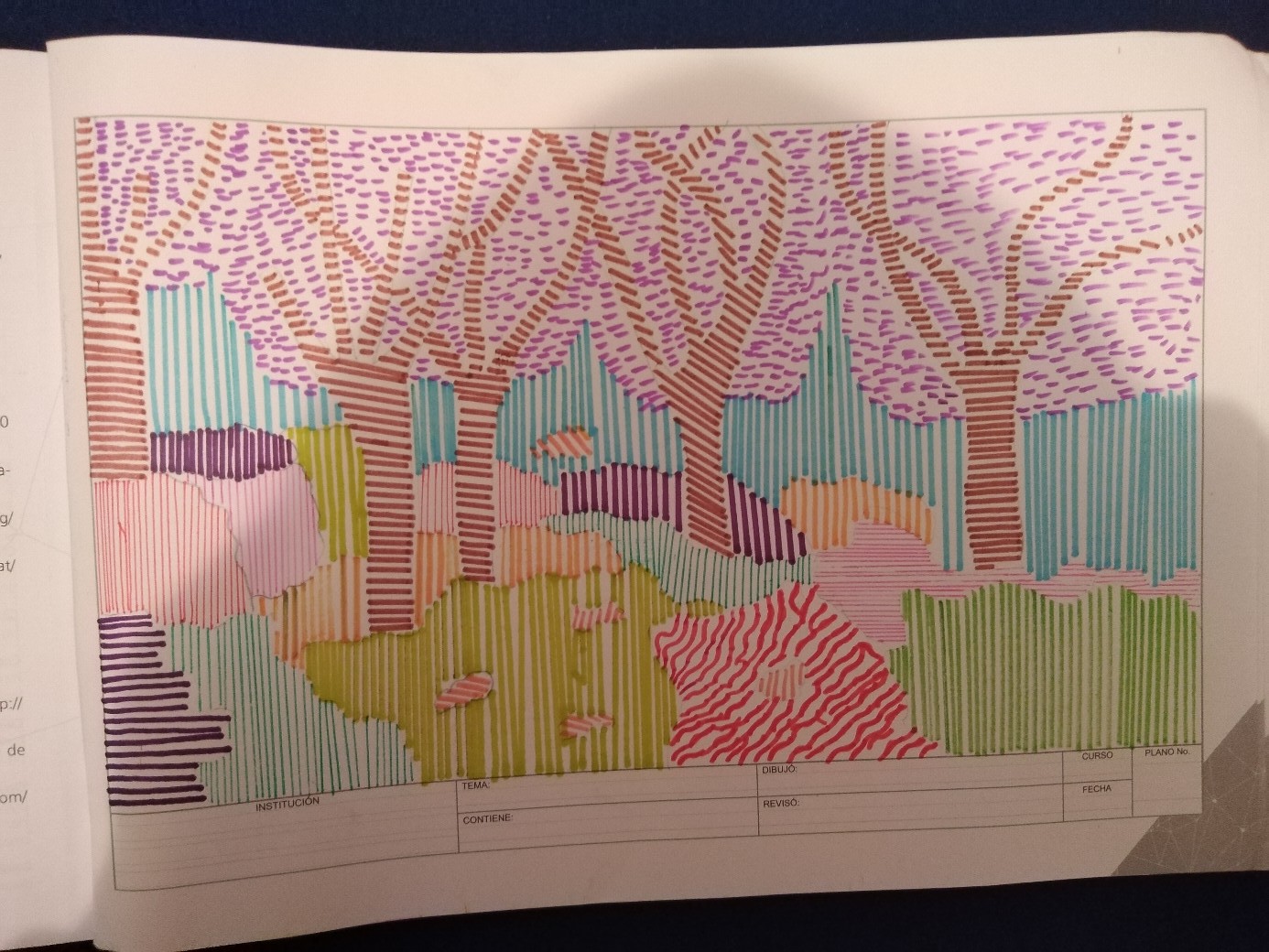This photograph captures a detailed drawing displayed on a black countertop, giving the impression of a page from a book. The paper is wide and horizontally oriented, revealing an open book with visible pages to the right and a noticeable crease to the left. The drawing itself is vibrant and colorful, featuring four distinct trees with purple canopies and straight-lined trunks in shades of brown. The ground beneath the trees is depicted with green grass, with patches of red and blue suggesting additional elements, possibly representing water bodies. Below the main illustration, there are several boxes likely intended for captions or additional text, though they are unreadable due to the low light and shadow cast over the majority of the page.